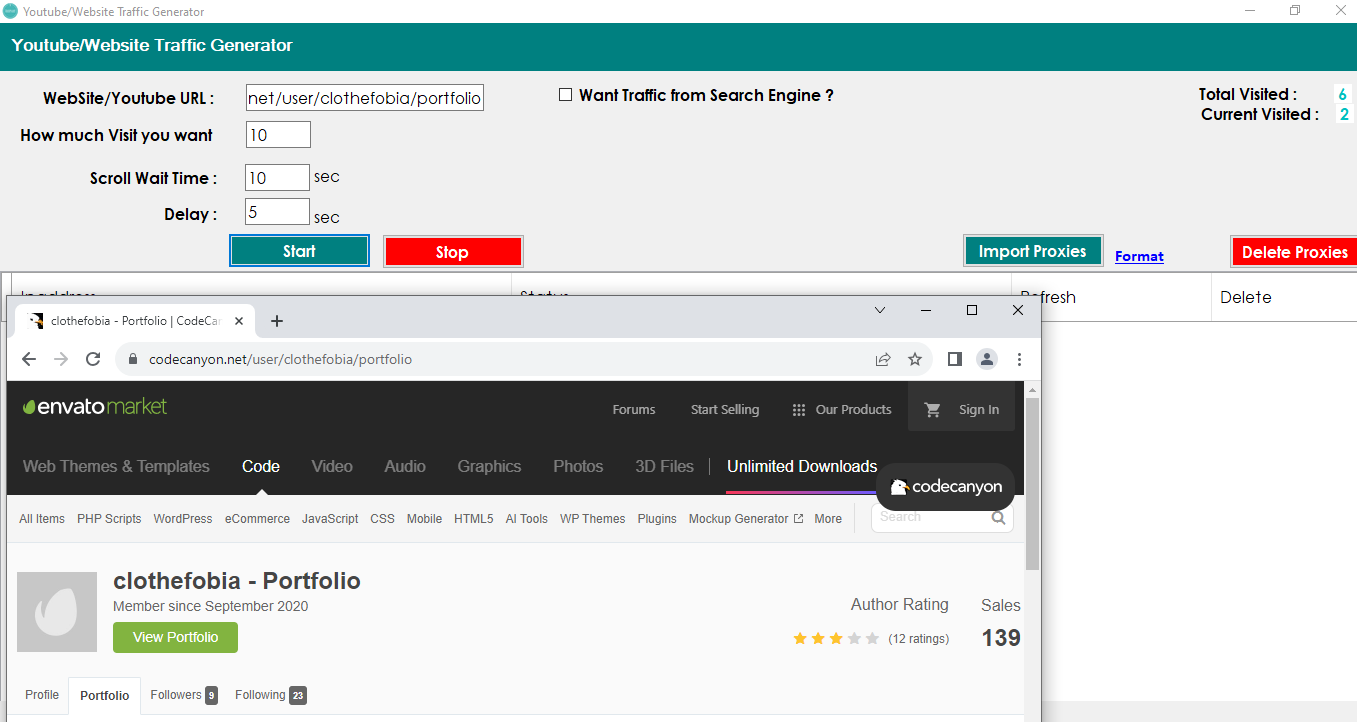A screenshot of an online tool for generating YouTube website traffic. At the top of the interface, there's a thin green strip with the text "YouTube Website Traffic Generator" in white. Below this, on a gray background, there's a text field labeled "Website/YouTube URL" containing the URL "net/user/cloth_ephobia/portfolio." Further down, there's a section labeled "How Much?" with a data field specifying "10" visits, a scroll time of "10 seconds," and an outside delay of "5 seconds."

Two buttons, "Start" (green with white text) and "Stop" (white with black text), are positioned below these settings. To the right, there's an option to check a box for "Traffic from Search Engines" with a question mark next to it. Further down, there are indicators showing "Total Visited: 6" and "Current Visited: 2" both in green. At the bottom, there’s a green "Import Proxies" button with white text, and next to it, a blue "Format" link, underlined for emphasis. On the bottom right, a red button labeled "Delete Proxies" in white text stands out.

Below the main interface, there is a tab that appears to be from the Envato Market website, indicated by the market’s branding - "Envato" in white and "Market" in olive green, with the URL "codecanyon.net/user/cloth_ephobia/portfolio" displayed in the address bar.